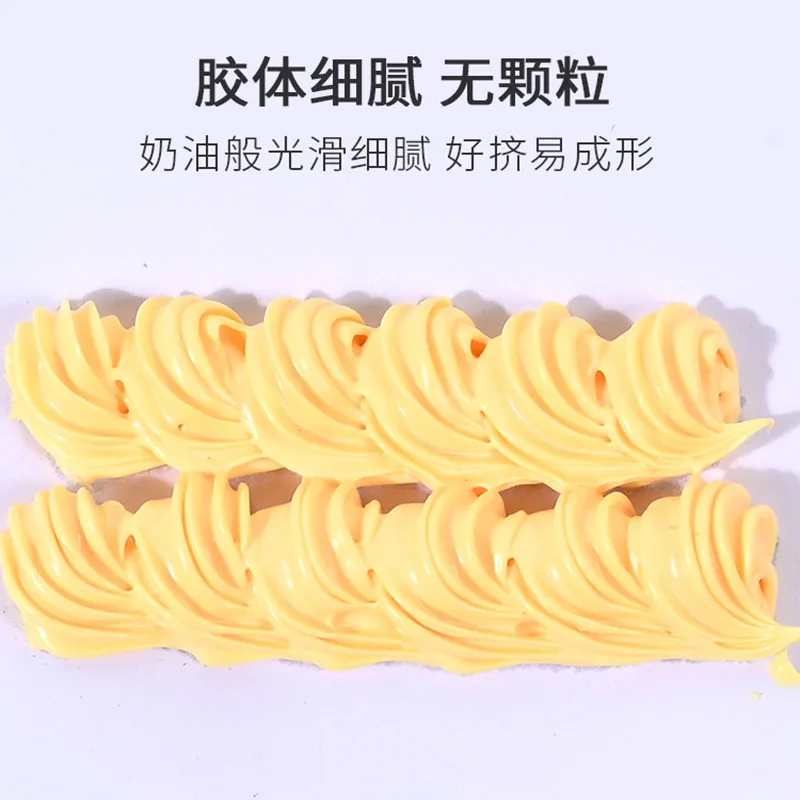This photograph features two rows of what appear to be large, swirled noodles or possibly an Asian treat, set against a pale light purple background. Each row contains six individual swirls, with the top row positioned directly above the bottom row. The swirls are a yellowish-beige color, glossy, and coated in what looks like cheese or frosting, with a texture reminiscent of seashells or piped cake frosting. Above the rows, there are two lines of bold Chinese text; the top line is thicker with around seven characters, while the bottom line is thinner and contains about 11 or 12 characters. The image, potentially an advertisement for these appetizing-looking noodles or treats, casts a slight shadow to the right, enhancing the three-dimensional appearance of the swirls.